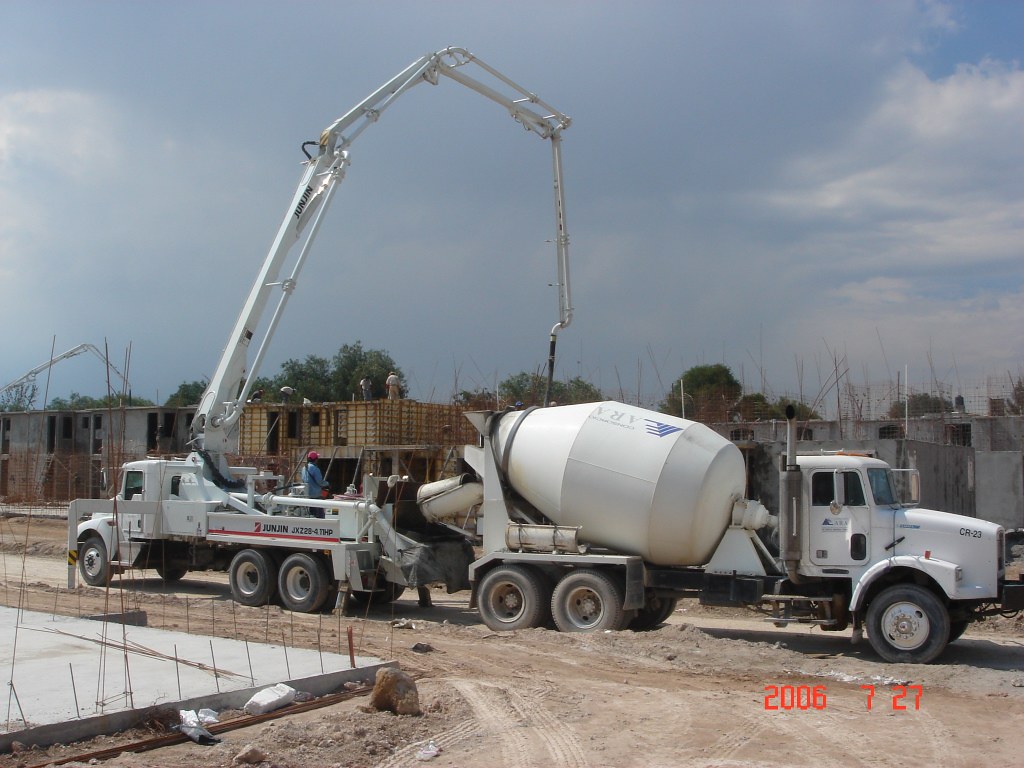This photograph, dated July 27, 2006, as noted by the red digital timestamp in the bottom-right corner, showcases a bustling construction site. In the foreground on the left, a considerable slab of freshly poured concrete features protruding rebar. Adjacent to this slab, a white cement mixer truck is actively engaged, its long hose apparatus stretching across the sandy, dirt-covered area akin to a crane as it channels cement towards various parts of the site. The crane-like structure appears to assist with moving materials or supporting the cement pumping process. 

In the background of the image, several two-story buildings are under construction, potentially apartments or houses. The skeletal structures of these edifices are partially revealed, with large wooden forms visible, perhaps for molding concrete. On a closer inspection, the absence of any visible human workers is notable, creating an almost eerie scene of automated labor in progress. The background reveals a mostly cloudy day, with a mix of white clouds and patches of blue sky, adding a subdued atmosphere to the industrious landscape. Overall, this photograph encapsulates a moment of dynamic building activity, underscored by the modern machinery orchestrating the development of new structures.